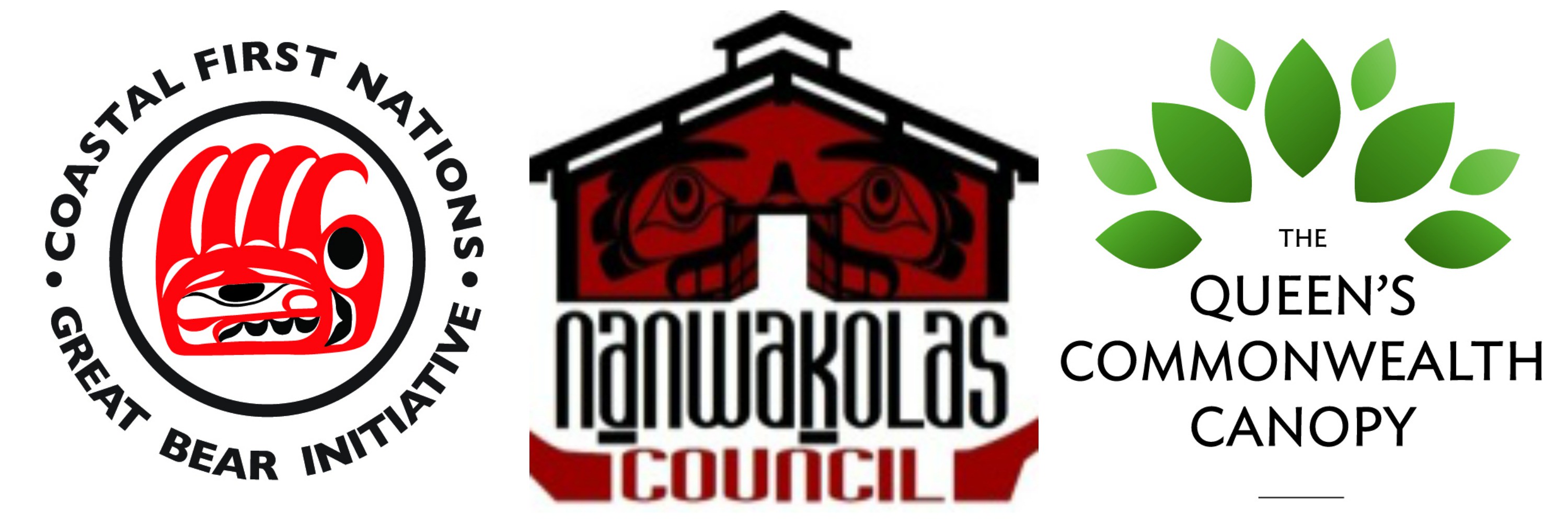The image features a collection of three distinct company logos, each set against an all-white background and evenly spaced in a horizontal arrangement, making them easy to see and distinguish. 

On the left, a circular logo for the Coastal First Nations Great Bear Initiative is displayed. This logo incorporates indigenous art, depicted with a simplified yet distinct black and red design, potentially representing a bear claw.

In the center, the logo for the Nanwakolas Council is showcased. It features an image resembling a barn with indigenous artwork that suggests facial elements, such as eyes, on either side of the structure. The logo text reads "Nanwakolas Council," spelled N-A-N-W-A-K-O-L-A-S.

On the right, the final logo is for The Queen's Commonwealth Canopy. It features a stylized plant or fanned-out leaf design, accompanied by the text "The Queen's Commonwealth Canopy."

The logos predominantly use colors like white, black, red, maroon, and various shades of green. The setting and style of these logos give the impression of professional business branding, possibly suited for company business cards.